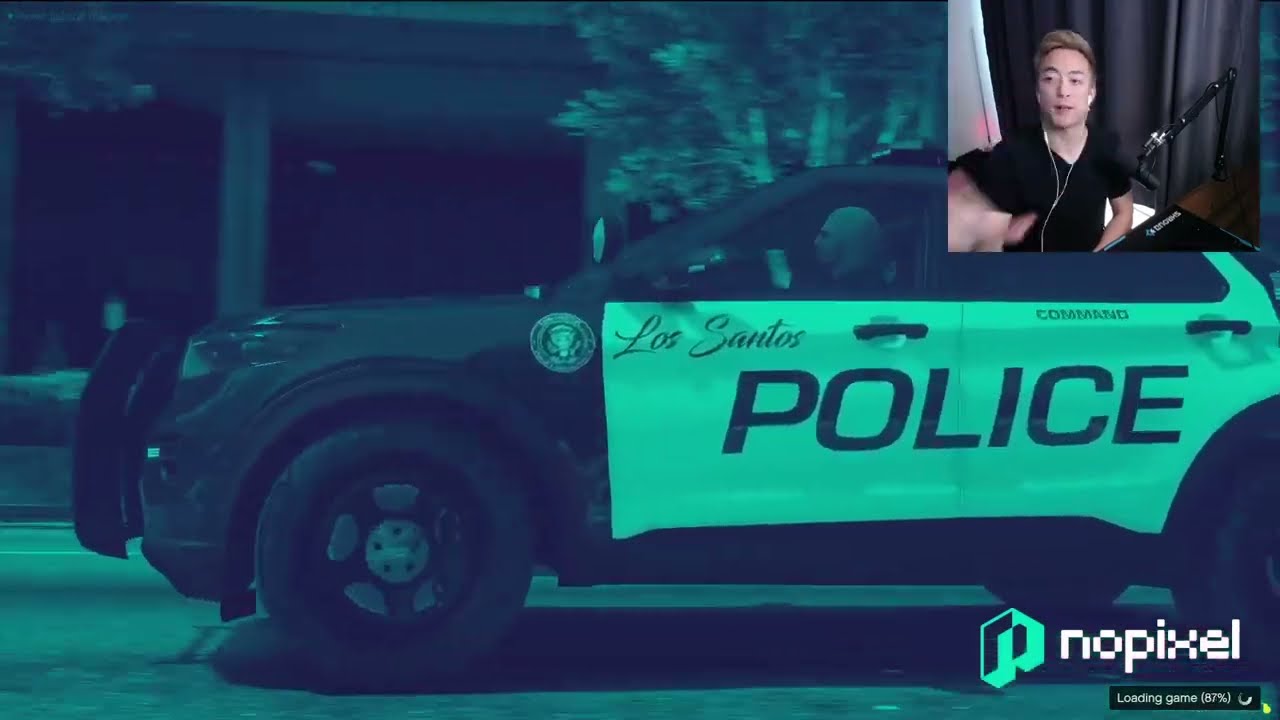The image depicts a loading screen from a video game, showing a Los Santos Police Department SUV, tinted with a washed-out greenish-blue filter that creates a black-and-white effect with a teal overlay. The police vehicle occupies most of the screen, oriented towards the left, with only the back tires partially visible. In the background, there's a city street with a sidewalk lined with a few trees and a storefront. In the upper right corner, a webcam feed of the gamer is visible, featuring a blonde-haired individual wearing a black shirt and white earbuds with a microphone. The gamer is situated in front of a heavy gray curtain, indicating he is engaging with the audience, possibly on a blog or streaming platform. The bottom right corner of the screen displays pixelated white letters that state "NoPixel," accompanied by a logo that resembles an "N" and the text "loading game 87%."